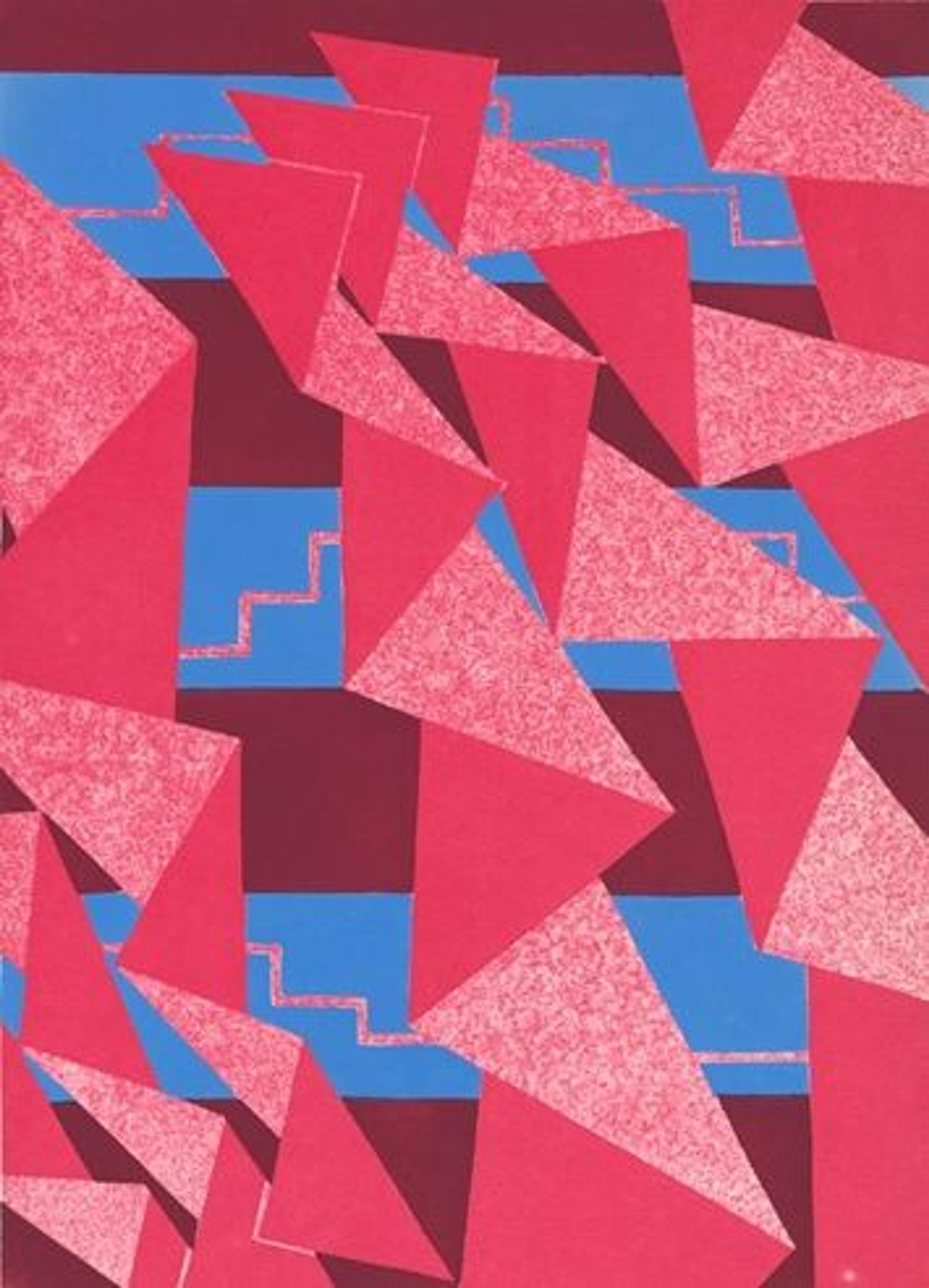The vertically-oriented, rectangular image showcases a vibrant geometric design on a burgundy background with three horizontal turquoise blue stripes positioned at varying intervals from the top, middle, and towards the bottom. The striking centerpiece of the image consists of origami-like folded paper structures in alternating two-toned shades of dark and light pink, arranged in a dynamic, zigzag pattern. These folded pink strands emerge from the bottom and are angled irregularly, with clusters prominently positioned in the lower left, upper right, and center of the image, creating a textured, origami-inspired effect. Alongside these elements, a grainy red and solid red stair-step pattern interweaves through the blue stripes, adding depth and complexity to the composition.